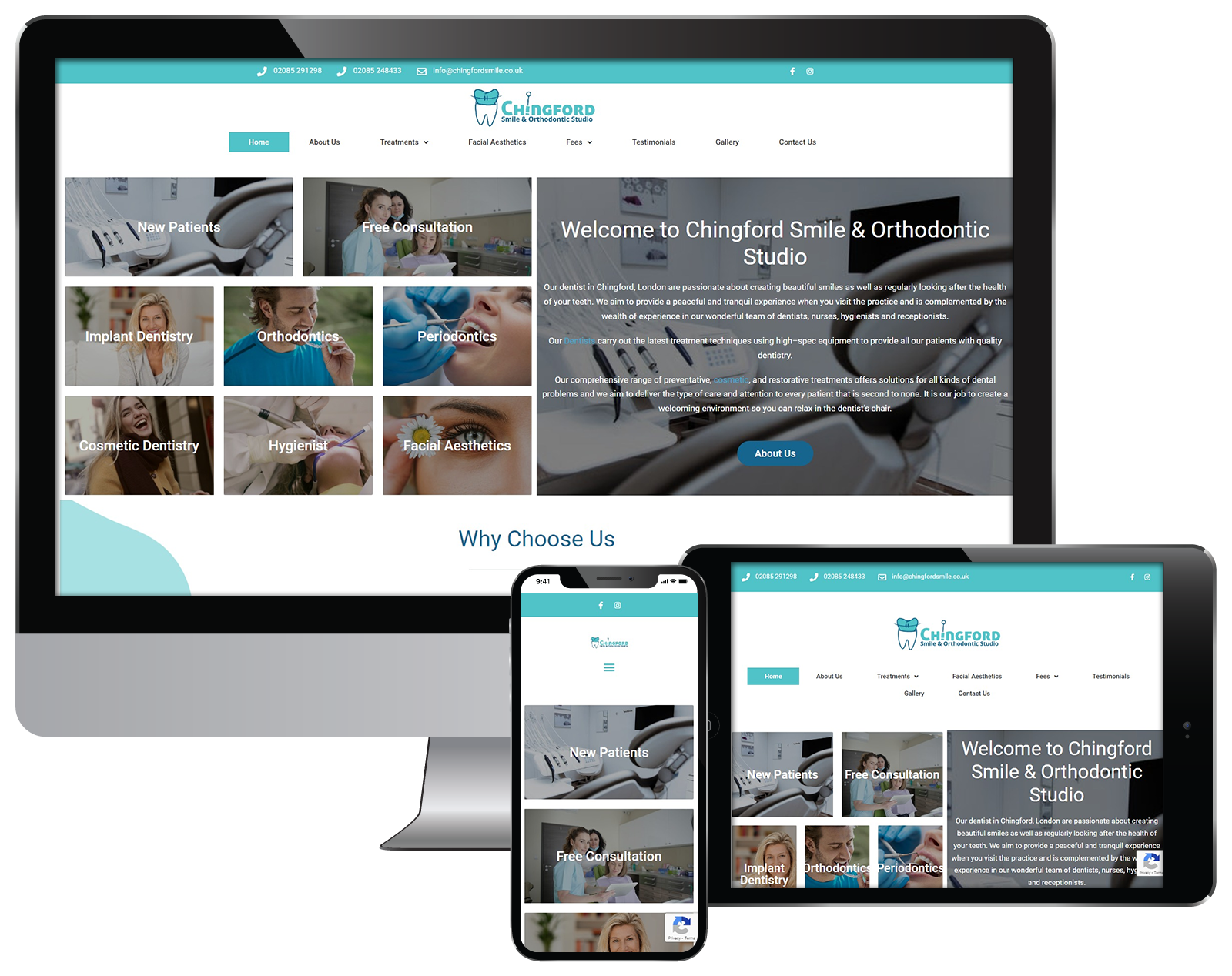The image depicts a flat-screen monitor, tablet, and cellphone, all displaying the same information from "Chingford Smile and Orthodontics." The top edge of the display is turquoise, featuring the text in white: "Phone: 020 8529 1298" and "Phone: 020 8524 8433." Additionally, the email address "info@chingfordsmile.co.uk" is listed.

On the right side of the display, there are Facebook and Instagram icons. The text "Chingford" appears in blue, followed by a turquoise and white tooth illustration. Below this, "Smile and Orthodontic Studios" is displayed in darker blue. All this information is set against a white background.

On the left side of the screen, a navigation menu is shown with turquoise buttons and white text, including options for "Home," "About Us," "Treatments" (with a dropdown menu), "Facial Aesthetics," "Fees" (with a dropdown menu), "Testimonials," "Gallery," and "Contact Us."

Below the menu, there are photo thumbnails with descriptive captions such as "New Patient Free Consultation," "Implant Dentistry," "Orthodontics," "Periodontics," "Cosmetic Dentistry," "Hygienist," and "Facial Aesthetics."